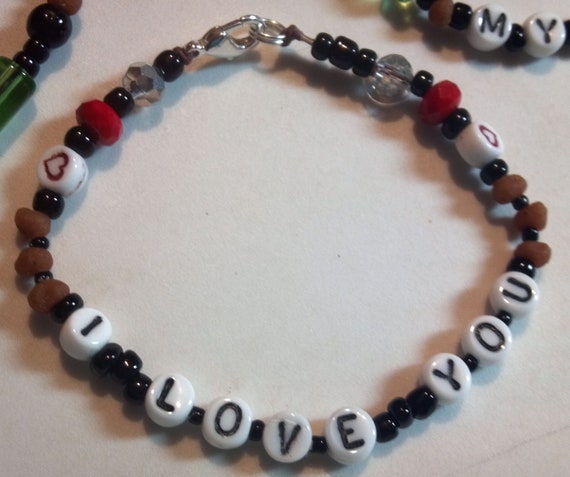The image depicts a handmade beaded bracelet sitting on a light tan countertop, designed with an array of colorful beads and detailed accents. Dominating the center of the bracelet is a sequential arrangement of white beads spelling out "I love you," each letter separated by a single black bead. The bracelet features an eclectic mix of bead shapes and sizes, including small round black beads, two large red beads, six brown pebble-like beads, and two clear crystal-like beads. Additional beads include white beads adorned with red heart symbols. The bracelet is secured with a silver clasp, hinting at either its handmade nature for selling or gifting purposes. Partially visible behind this focal piece are two other bracelets; one reads "my," while the other is characterized by a green clasp and black beads. The entire set of jewelry rests on a cream-colored surface, promising to catch the eye of anyone who might appreciate its intricate and heartfelt craftsmanship.